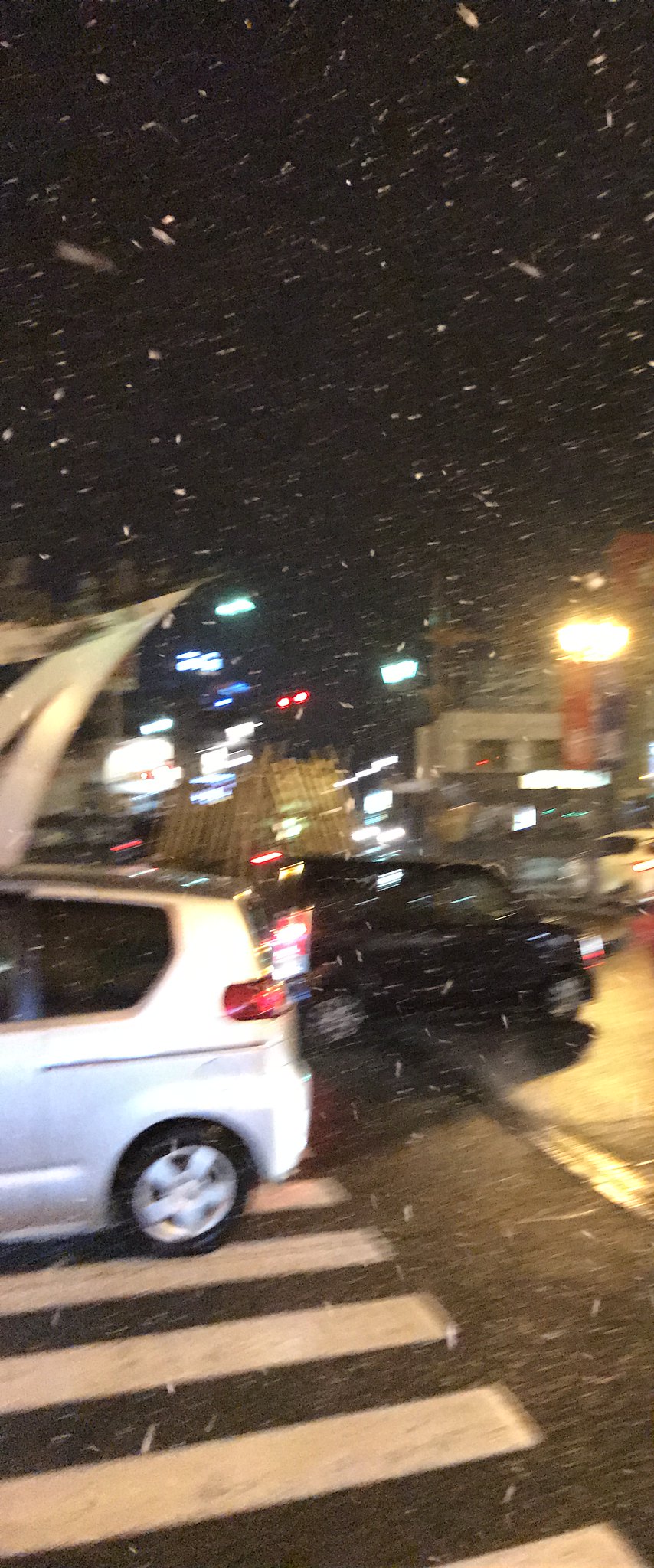The image depicts a nighttime scene of a parking lot lightly dusted with the initial downpour of snow. Large, distinct snowflakes fall from a dark sky, creating an array of sparkling particles that enhance the wintry atmosphere. The ground, however, is yet to be covered, signaling the beginning of the snowfall. In the parking lot, a silver compact SUV is parked head-in on the left side of the frame, while on the right, a black SUV faces the opposite direction. The cars are strategically placed within rectangular parking spaces that are uniformly marked. Illuminating the scene are various light sources, including street lights, traffic lights, and the glowing lights from distant buildings, all creating a blurred and muted blend of whites, greens, blues, and reds. Additionally, there is a striking contrast between the black asphalt of the crosswalk and its prominent white lines, which are noticeable amidst the gently falling snow. A bamboo fence can also be seen in the background, adding a touch of texture to the urban locale.